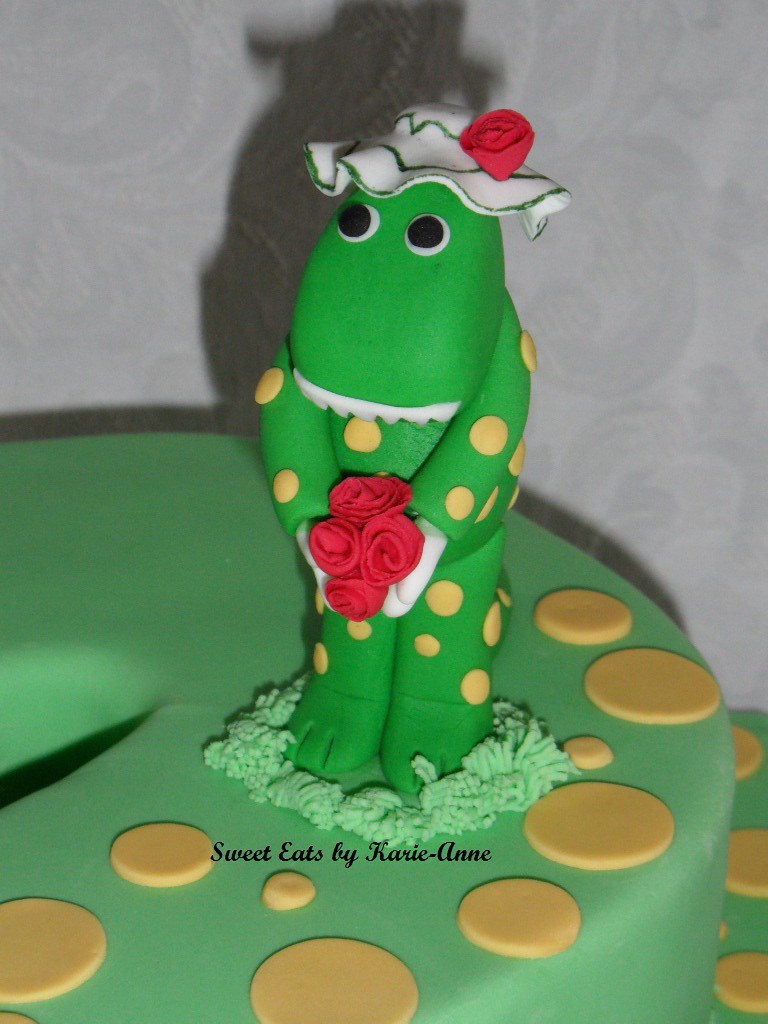The image showcases a detailed close-up of a two-tiered cake, with a predominant focus on the top tier. The cake is covered in a light green fondant and decorated with various sizes of light yellow dots scattered across its surface. The most striking feature is the cake topper, which depicts a whimsical frog character. This frog, matching the green of the cake with yellow polka dots, stands upright and wears a white sun hat adorned with green stripes and a single red rose. It has large white eyes with black pupils and holds a bouquet of five red roses in its hands. The figure's feet appear to be surrounded by a texture resembling green grass. The cake is further personalized with an overlay of black text in small font below the topper, reading "Sweet Eats by Carrie Ann."